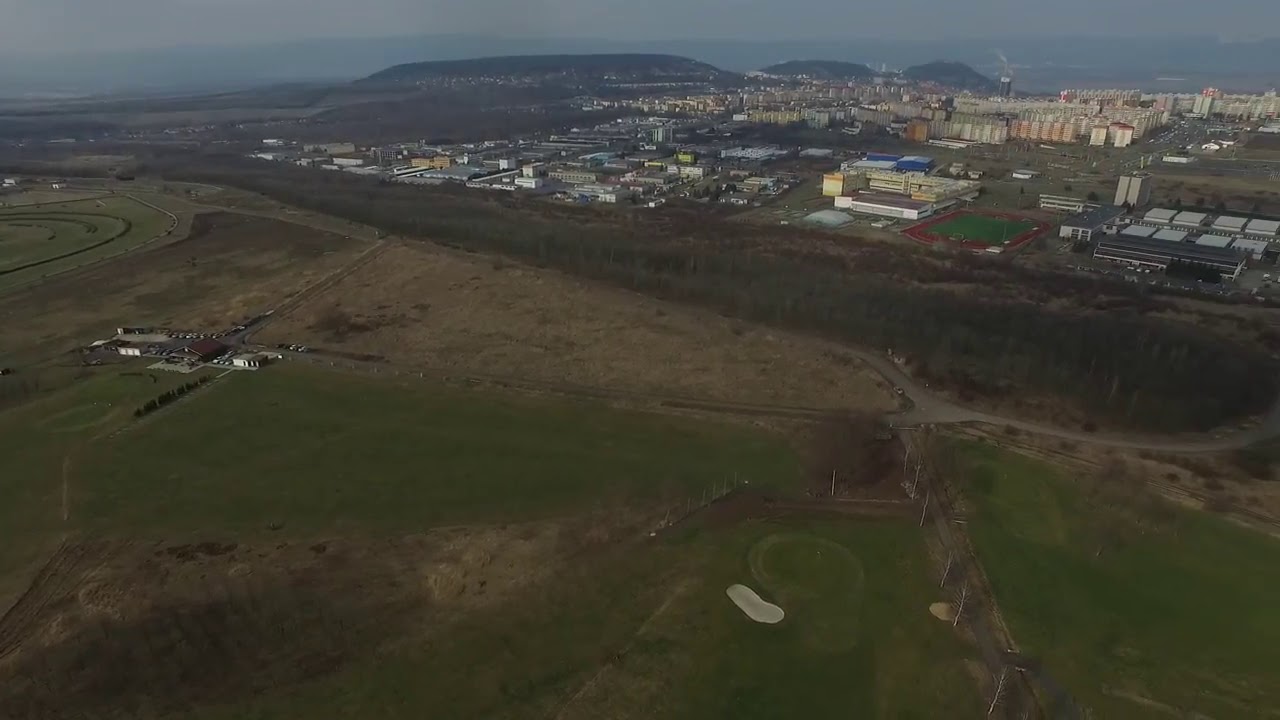The image presents a detailed aerial view of a landscape with distinct sections of rural and urban areas. In the foreground, there's a predominantly flat expanse of undeveloped land and farmland. This area features a notable small forest segment emerging from the bottom left corner, framed by surrounding grassland. Connecting roads traverse the fields, leading towards the upper section of the image.

Beyond the farmland, there's a substantial strip of land that appears swampy, serving as a transition zone between the rural expanse and the more urbanized part of the scene. This intermediary area is highlighted by a thin line of trees, effectively segmenting the landscape. In the upper part of the image, most of the buildings cluster, showcasing a mix of towering skyscrapers and industrial-type structures, giving the sense of an industrial district. 

To the right, there is a distinct sports field that resembles either a baseball or football field. In the far background, distant hills or mountains outline the horizon, with a possible glimpse of water to the right, adding depth to the scenery. Overall, the image juxtaposes the tranquil, open fields and forested areas of the foreground with the bustling urban landscape and industrial buildings beyond, framed by natural features like hills and water.